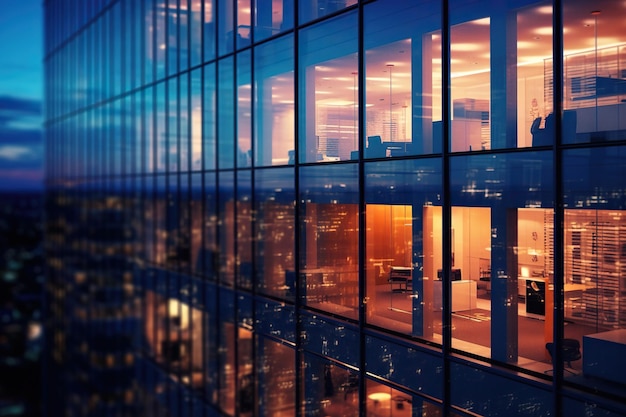The image depicts a high-rise glass office building at dusk, set against a night sky tinged with dark blues and purples. The side perspective reveals furniture inside the illuminated rooms, casting a warm golden, amber hue. City lights from surrounding skyscrapers reflect off the glass facade, creating a complex pattern of light and shadows. Through the windows, various office furnishings are visible, including desks, chairs, tables, and possibly kiosks or long poles. Some windows have shutters, and one desk appears to have a black object on it. The photo captures a few floors of the building, emphasizing the office spaces that extend into the distance.